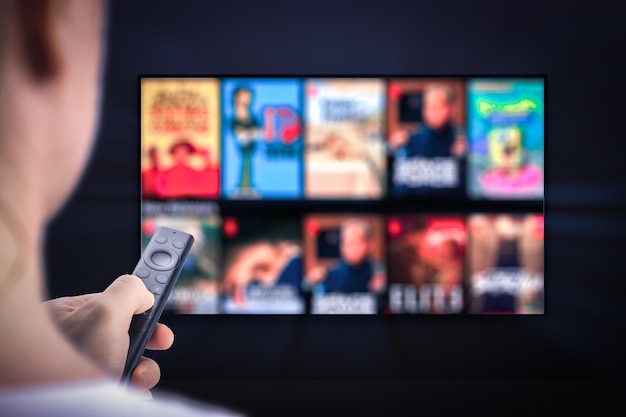In this image, we see a person interacting with a streaming service interface. The individual, whose blurred figure is positioned in the left foreground of the photo, grips a sleek, black smart remote in their left hand. Their thumb hovers over the central button of the remote, poised to either make a selection or navigate through the options. The room appears dimly lit, contributing to the overall dark ambiance of the scene. 

In the background, a television screen displays a menu with ten blurred show or movie titles. Among these, the only discernible title is "SpongeBob SquarePants," located in the upper right corner. The interface suggests a streaming service, possibly Netflix, as indicated by the familiar red tag in the upper left corner of the thumbnails, which often denotes popular content. The majority of the background is indistinct, emphasizing the remote and the act of selection as the primary focus of the image.